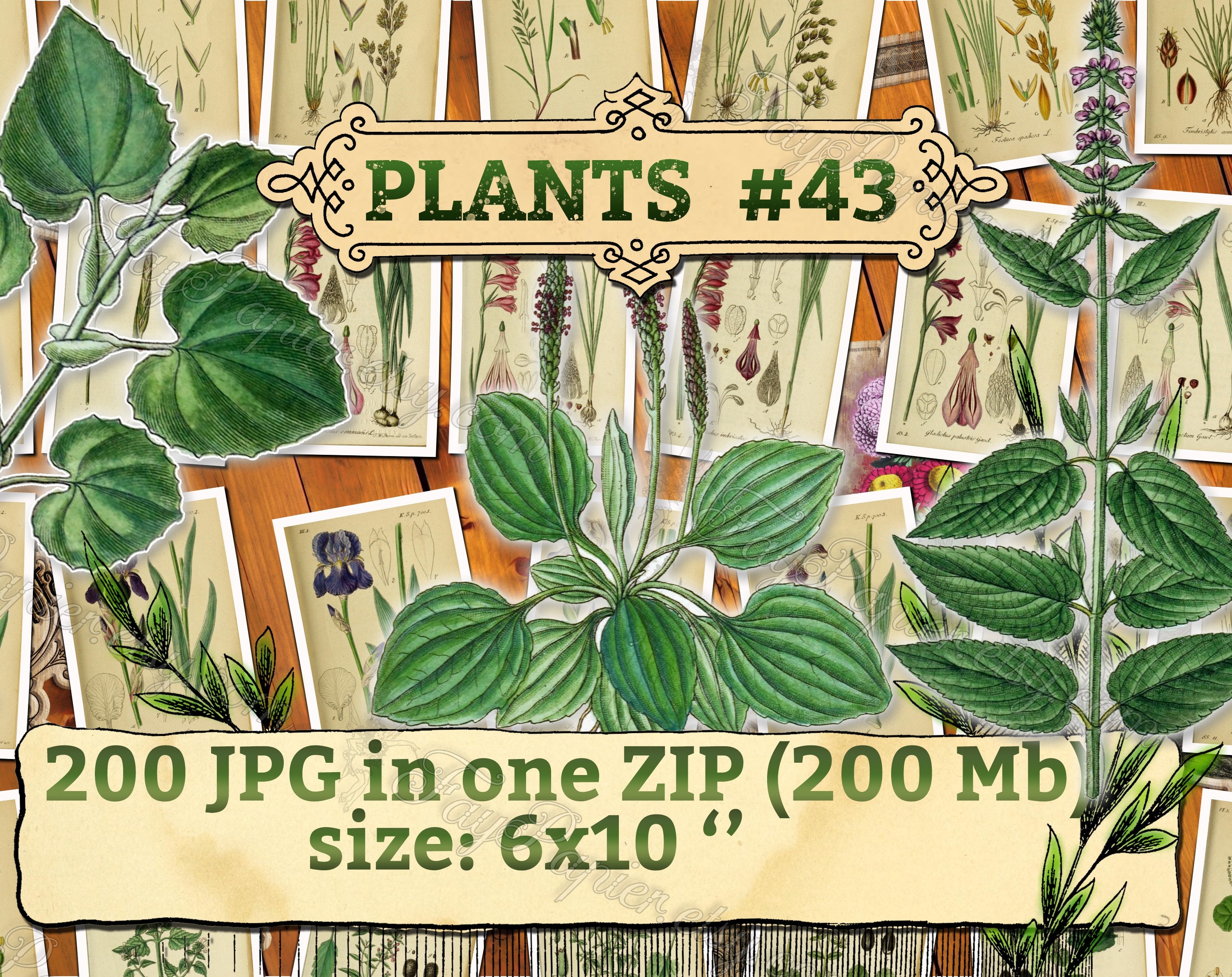This image appears to be an advertisement for a digital product, specifically a collection of plant-themed illustrations. The focal point at the top is an ornate text panel labeled "Plants Number 43" in green font over a beige background, adorned with stylized squiggles at the top, bottom, left, and right. Below this heading, the central area features three lush green plants with broad leaves, two of them bearing purple flowers. Complementing this are arrays of painted, animated leaves scattered throughout the image, creating a vibrant background. Interspersed among the leaves are various cards or envelopes depicting different plants and flowers, each with white borders and taupe backgrounds, all set against a flat wooden surface.

Near the bottom of the image, an off-white banner clearly states in green text: "200 JPG in one ZIP (200 MB), size 6 by 10 inch." This indicates the digital product offered is a zip file containing 200 high-quality JPG images, totaling 200 megabytes in size, with each image sized at 6 by 10 inches. The overall green theme, due to the abundance of plant illustrations, creates a cohesive and visually appealing advertisement for the collection.